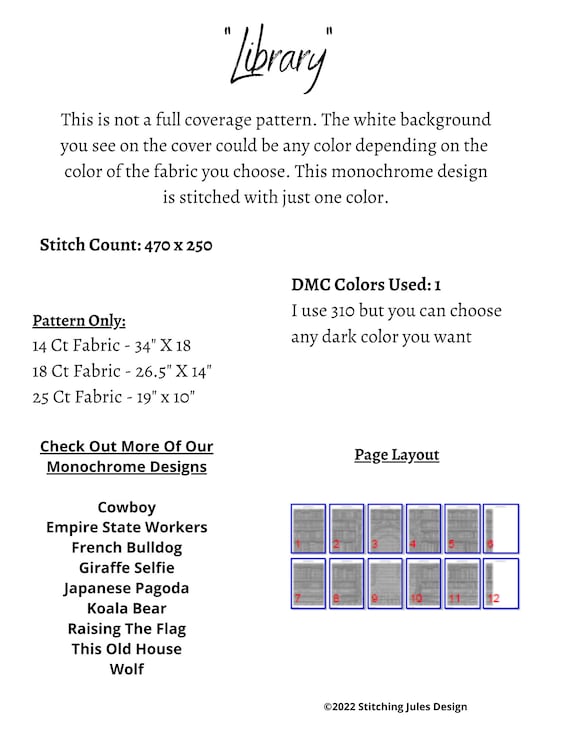The image depicts a detailed white page with dense black text and a diagram at the bottom. The top of the page features the word "Library" in a cursive-like script enclosed in quotation marks. Below this, it indicates that this is not a full coverage pattern and emphasizes that the white background can be any color, depending on the fabric chosen. The monochrome design is to be stitched with just one color. Further down, it specifies a stitch count of 470 x 250.

On the right side near the top, bold text reads "DMC Colors Used: 1," with a note stating, "I used 310, but you can choose any dark color you want." To the left, it mentions "Pattern Only" and lists yardages for different fabric counts, including 14, 18, and 25 count fabrics.

Beneath this, a section encourages checking out more monochrome designs, listing titles such as Cowboy, Empire State Workers, French Bulldog, Giraffe Selfie, Japanese Pagoda, Koala Bear, Raising the Flag, This Old House, and Wolf. Further down on the right, the page layout is detailed, showing 12 numbered panels, where most are shaded in gray except for two on the right vertical column. 

At the bottom, in fine print, the page states, "Copyright 2022 Stitching Jewels Design."